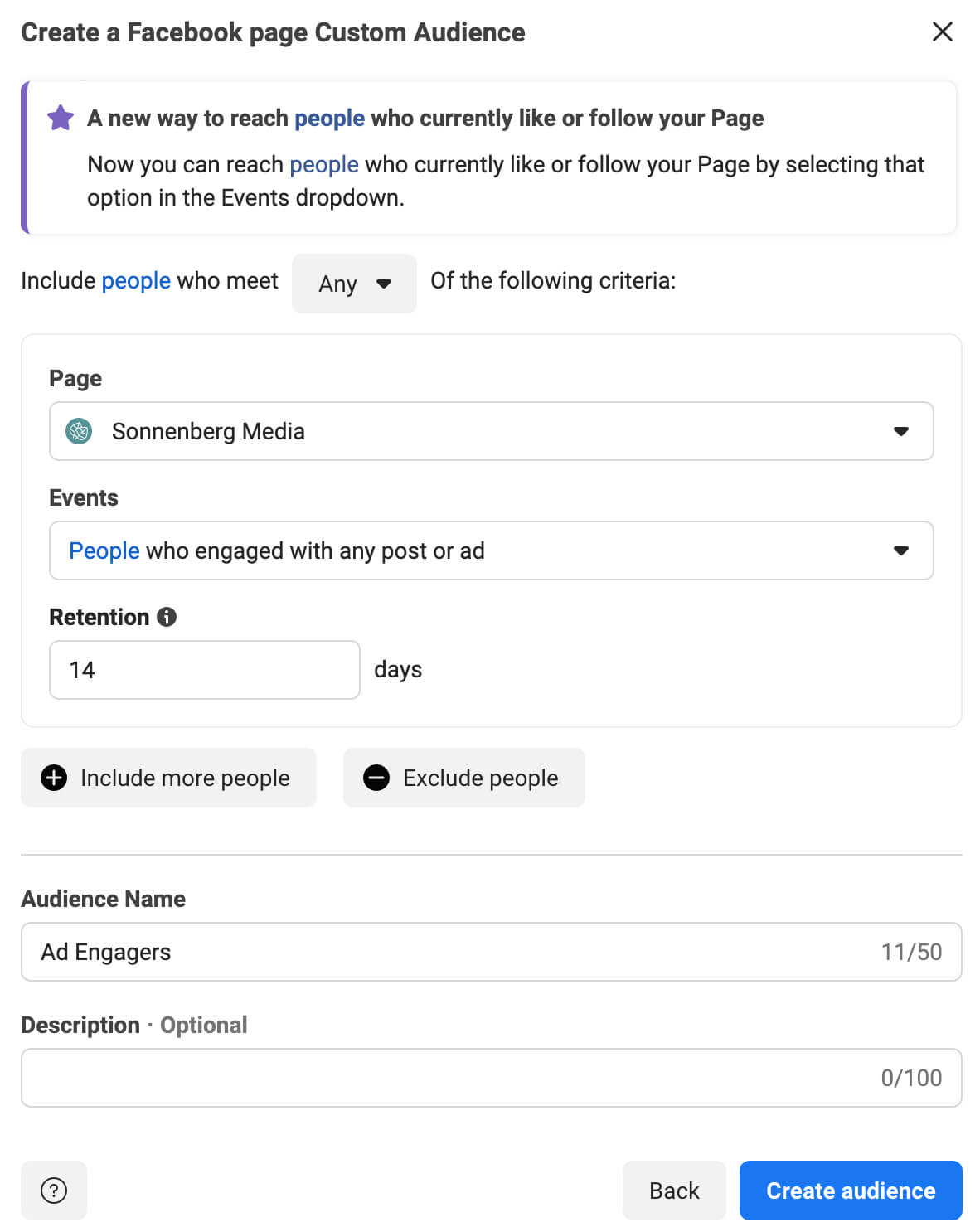The image is a detailed screenshot of a Facebook interface for creating a custom audience. The background is entirely white, making the black text at the top stand out. The text reads, "Create a Facebook Page Custom Audience." Below this heading, there's a pop-up box with the message, "A new way to reach people who currently like or follow your page. Now you can reach people who currently like or follow your page by selecting that option."

In the 'Events' dropdown, a purple star icon is positioned next to the text. The word "people" appears twice, both instances being blue hyperlinks. Moving down, there's a segment that reads "Include people," with the word "people" hyperlinked again. It continues with, "that meet any of the following criteria," accompanied by a grey dropdown menu.

Below this section, a white box is displayed featuring the word "Page" next to a dropdown menu that lists "Sonnenberg Media," identified by a green logo on the left side. Underneath this, the text reads "Events: People who engaged with any post or ad." Further down, there's a section labeled "Retention," which mentions "14 days."

At the bottom of the interface, options to "Include More People" or "Exclude People" are provided. Finally, there are fields labeled "Audience Name" and "Description (Optional)," with the values "Ad Engagers" (11 out of 50 characters used) and the description field showing "0 out of 100" characters used.